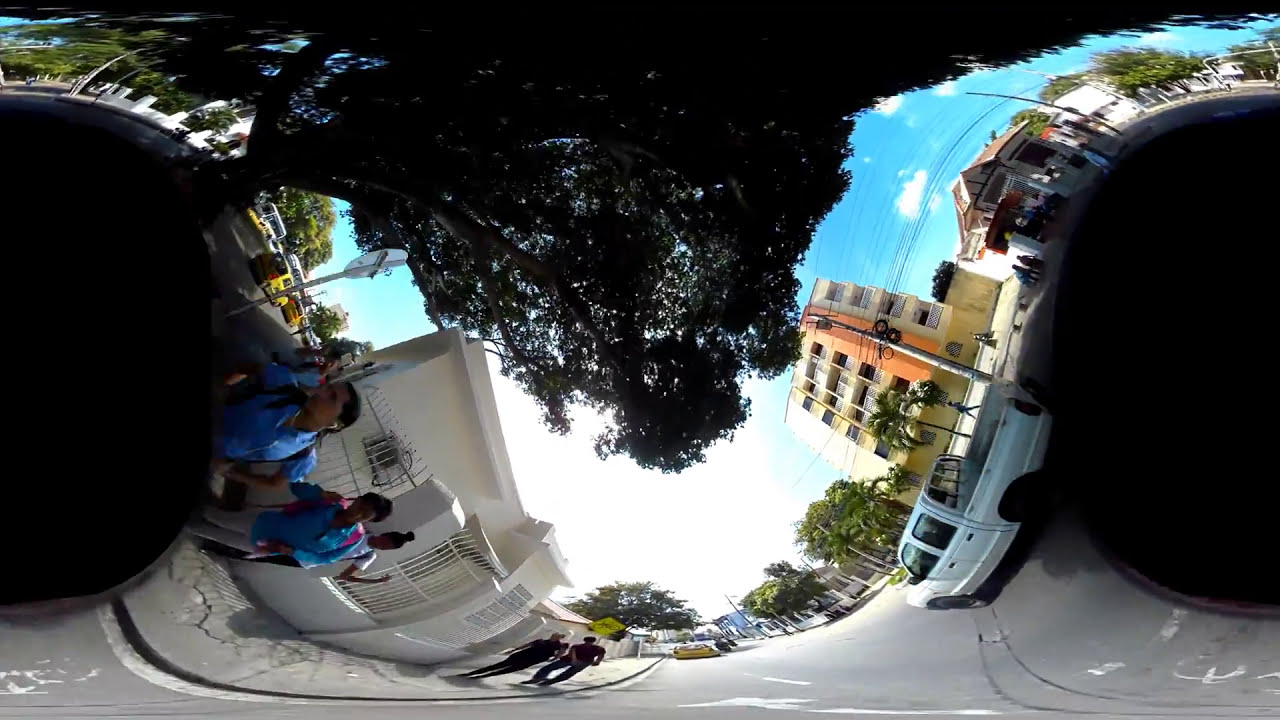This photograph showcases a heavily distorted street scene, seemingly taken with a panoramic lens. The image is marked by two conspicuous black regions on either side, creating a "black hole" effect. In the foreground on the left, a group of individuals wearing blue tops, possibly schoolchildren, are gathered on the sidewalk. Slightly further back, in the center of the image, two people dressed in black are walking toward the camera. To the right, a white truck is in motion while other vehicles are parked along the distant left side of the street. The street itself separates a yellowish-orange building on the left from other structures, including a prominent white building and an apartment building on the right. A bright blue sky with scattered white clouds and the presence of palm trees and power lines add to the suburban atmosphere. Despite the warping effects, the elements of daily urban life—buildings, vehicles, and pedestrians—remain discernible.